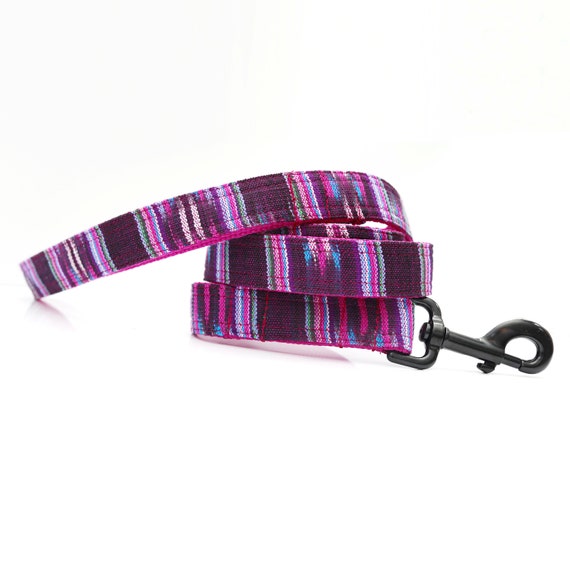The image displays a dark purple lanyard with lighter purple stripes, meticulously coiled into three loops, resting on a stark white background. This lanyard, fashioned from fabric, features diverse colors, including magenta accents and various stripes in shades of pink, burgundy, light blue, light green, and white, creating a vibrant pattern. On the right side, there is a shiny black plastic hook, which serves as a clasp for the lanyard.